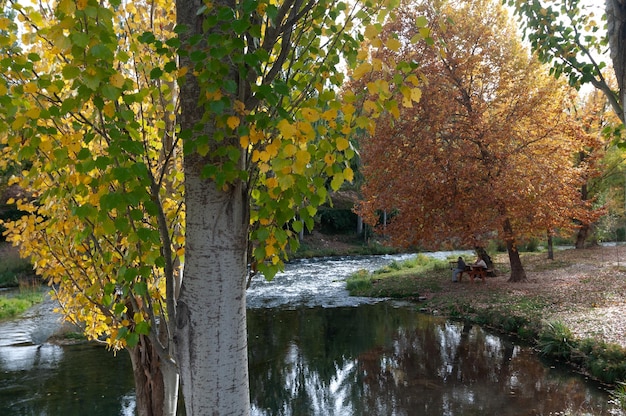In a picturesque autumnal scene, a serene stream meanders through a small forested park area, transitioning from foamy white water in the middle distance to a smooth, calm pond nearer the viewer. Multiple trees are scattered across the landscape, their leaves a vibrant mix of yellow, orange, and green. On the left side, a tree with half its leaves green and yellow stands visibly. On the far side of the stream, a tree with predominantly orange leaves is leaning toward the water, looking ready to shed its foliage. Underneath this tree, a picnic bench supports two people who appear to be enjoying the tranquil setting, while elsewhere a man in blue sits with a brown dog beside him. The ground is littered with dead leaves, and in the upper right corner, the sky is adorned with white clouds, completing this idyllic autumn day captured in full color.